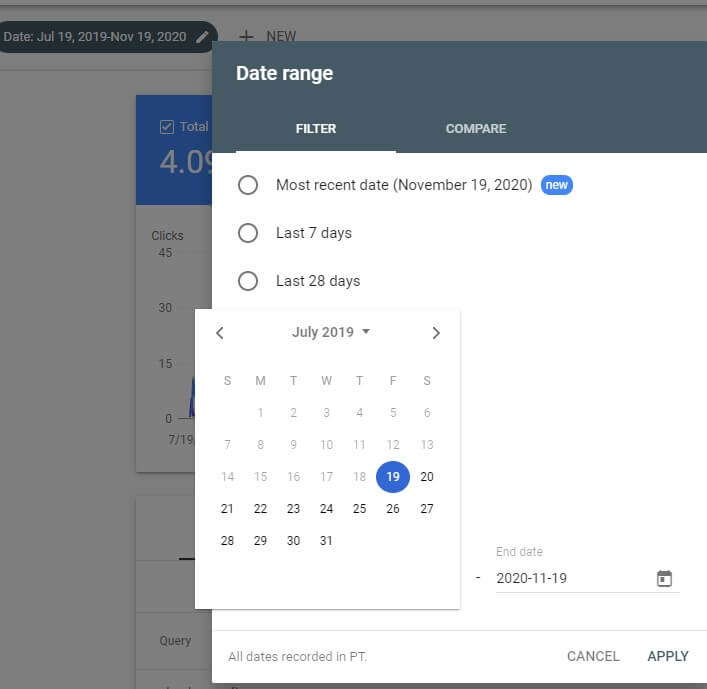The image portrays a screenshot of a date range selection interface, likely part of a web analytics or reporting tool. The interface is divided into two primary tabs at the top, labeled "Filter Active" and "Compare." The currently observed date range extends to the most recent date, November 19, 2020, marked with a "New" tag. Preset date ranges such as "Last 7 days" and "Last 28 days" are also available for quick selections.

A calendar dropdown is expanded, displaying the month of July 2019, with the selected date highlighted as July 19, 2019. Navigation arrows on either side of the displayed month facilitate switching between different months. The end date is set as November 19, 2020, mistakenly referred to as October 19, 2020, within the text. All dates are recorded in Pacific Time (PT).

At the bottom of the interface are the "Apply" and "Cancel" buttons, enabling the user to confirm or discard their date range selection. The layout supports the facile selection of predefined date ranges or allows the user to manually choose a specific range via the calendar interface. The active "Filter" tab implies that the user is configuring data filters to search, analyze, or view particular data segments.